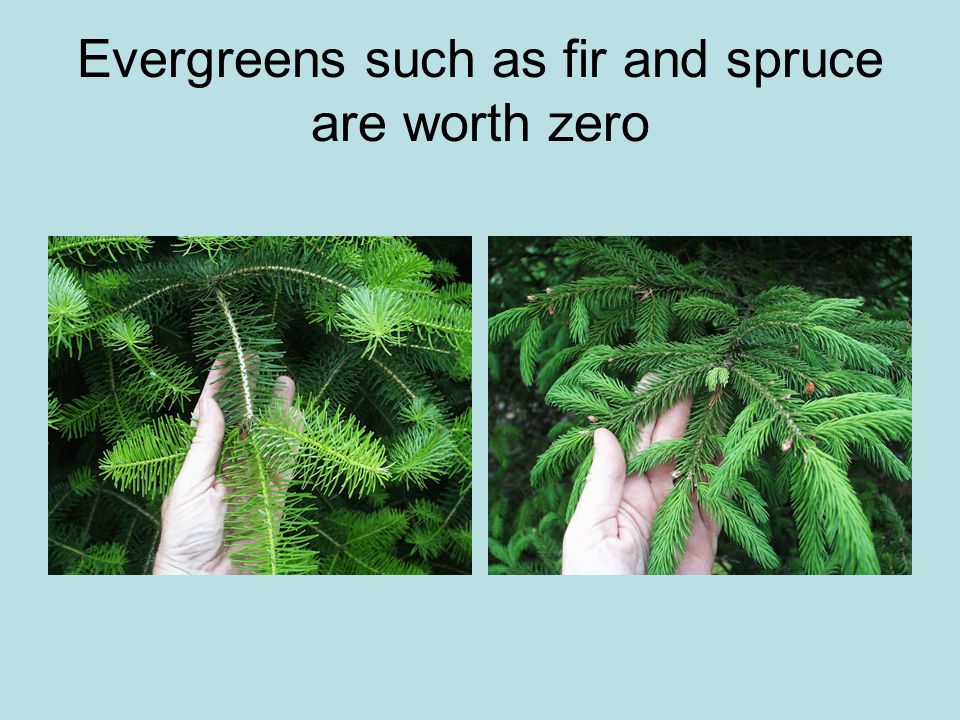The image is a digital collage featuring two square photos side-by-side, set against a light blue-green, almost teal background. At the very top, in plain black Times Roman font, is the caption: "Evergreens such as fir and spruce are worth zero." In the left photo, a pale, slightly wrinkled hand holds a lighter green plant assumed to be a fir, with pronounced white or light green spines and small, thin leaves. Surrounding this plant are similar green leaves suggesting it's part of a bush or larger plant. In the right photo, the same hand, now open and flat with fingers barely visible except for a thumb, holds a slightly darker green plant, likely a spruce. This plant has less noticeable spines and more clustered leaves, with a long leaf extending diagonally downward. The background shows shadowed plants that resemble clovers, and the overall scene is minimalistic, focusing solely on the hands and plants.